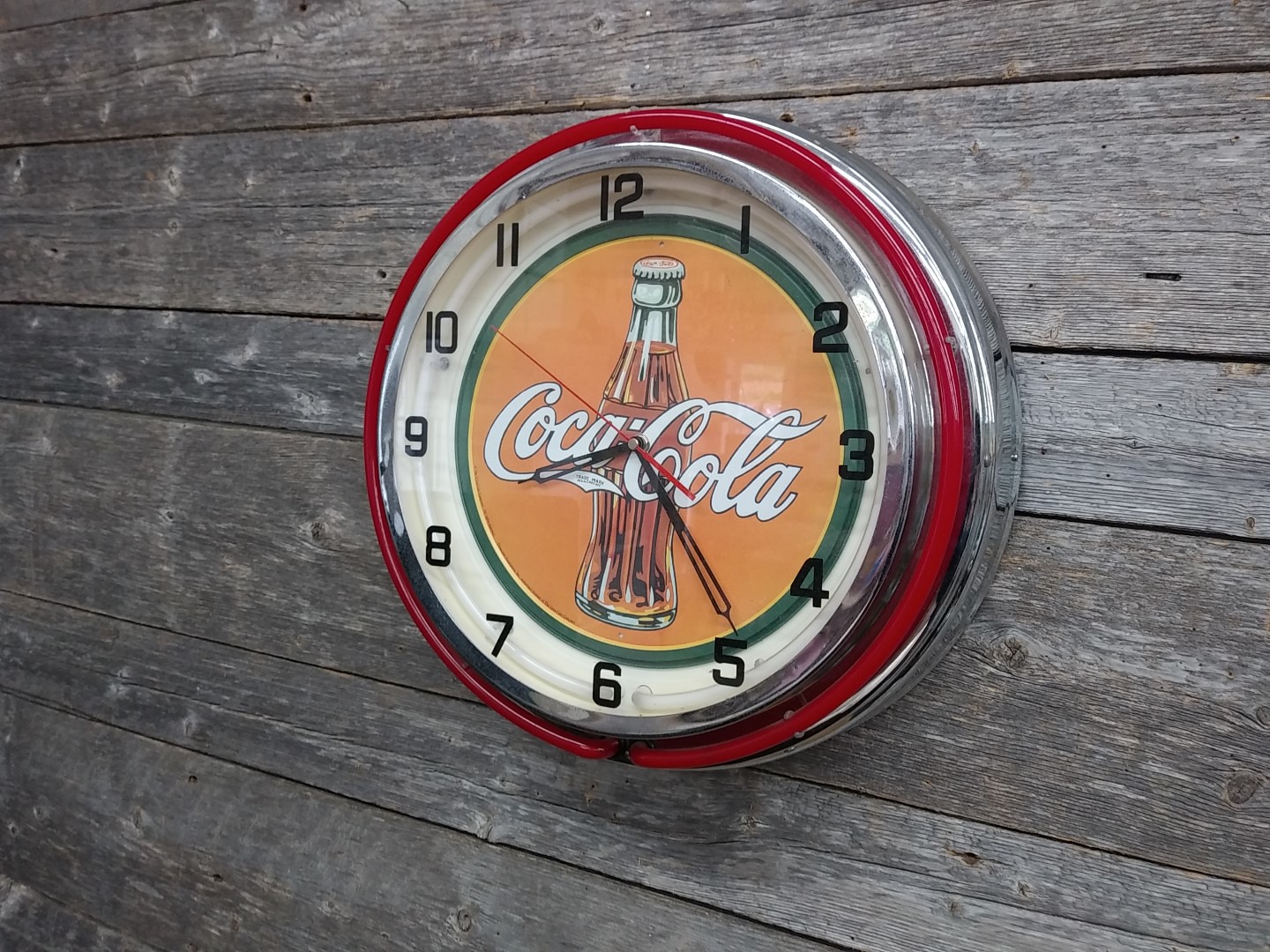The image features an old, weathered wall composed of horizontally aligned wooden slats that range in width from narrow to wide, and display varied shades of gray and brown, marred by white and black spots of age and dirt. Mounted on this aged wall is a distinctive Coca-Cola clock. The clock boasts an outer frame that appears to be a shiny chrome metal, adorned with a red border that resembles a neon light, although it is not illuminated in the daytime shot.

Inside the chrome frame is a glass casing, upon which the numbers 1 through 12 are painted in black. The clock face itself includes a cream-colored circle encircled by a green border, with an orange background at its core. The iconic Coca-Cola script, written in white letters, occupies the center, accompanied by an illustration of a classic curved Coca-Cola bottle.

The clock’s time reads 8:24, with the hour hand pointing at the 8 and the minute hand at the 5, while the thin red second hand is around the 52-second mark. This combination of elements creates a vivid, nostalgic depiction of the Coca-Cola brand against a backdrop that underscores the passage of time.